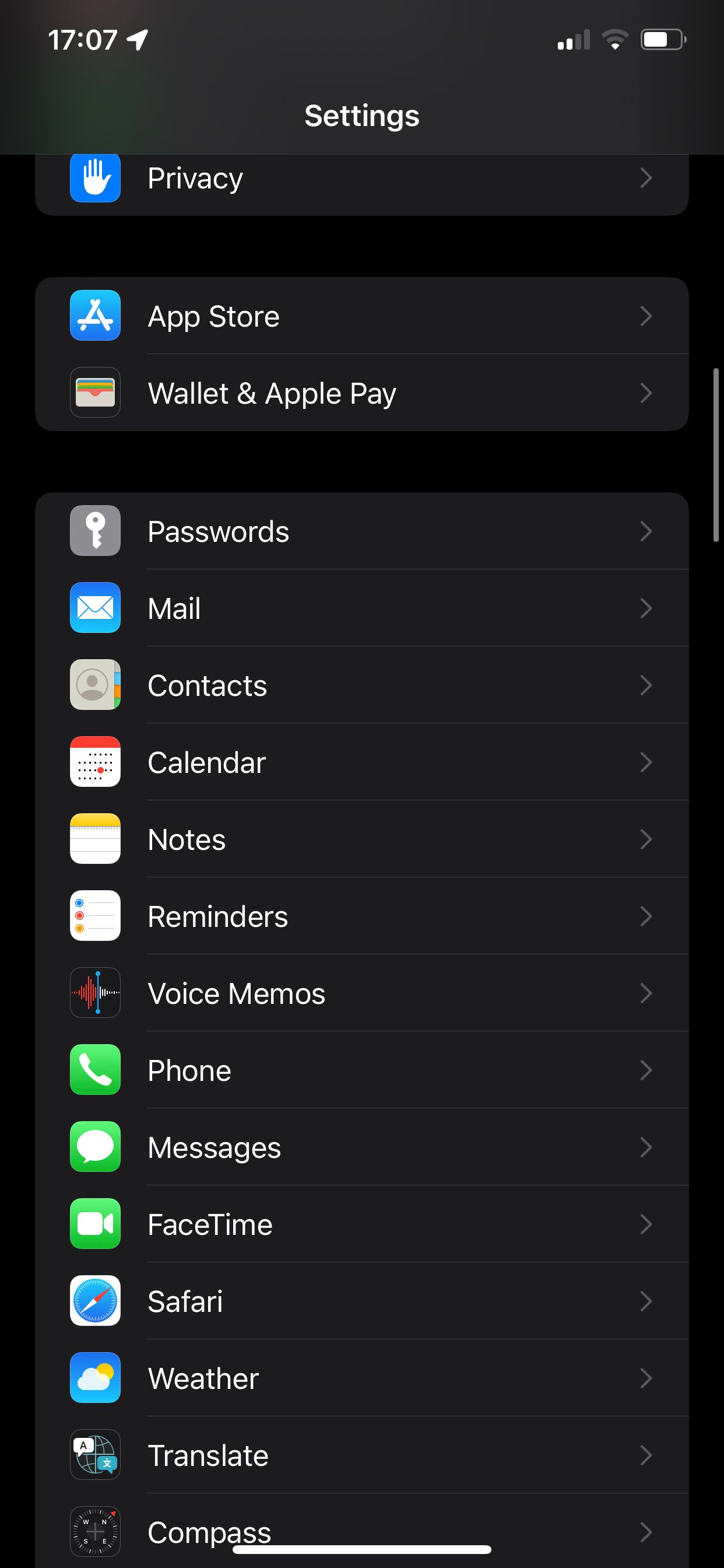This is a screenshot of a mobile device's settings panel. At the top left, the current time is displayed, followed by a location icon to its right. On the right-hand side, the icons for signal strength, WiFi connectivity, and battery status are visible. Centrally positioned below these icons, the word "Settings" is prominently displayed in white font.

Directly beneath this heading, the settings categories are listed. The first category is "Privacy," accompanied by an arrow on the right, indicating that it can be expanded to access more options. Following "Privacy," the list includes "App Store" and "Wallet & Apple Pay," each also marked with arrows to the right for further navigation.

Further below, the panel continues with a longer vertical list of additional settings categories, some housed within a lighter-colored block for distinction. Each category features a corresponding thumbnail icon on the left, the category title to its right, and an arrow on the far right, signifying expandability. The categories visible in this section include "Passwords," "Mail," "Contacts," "Calendar," "Notes," "Reminders," "Voice Memos," "Phone," "Messages," "FaceTime," "Safari," "Weather," "Translate," and "Compass."

This detailed and structured layout allows users to easily navigate and customize their device settings.